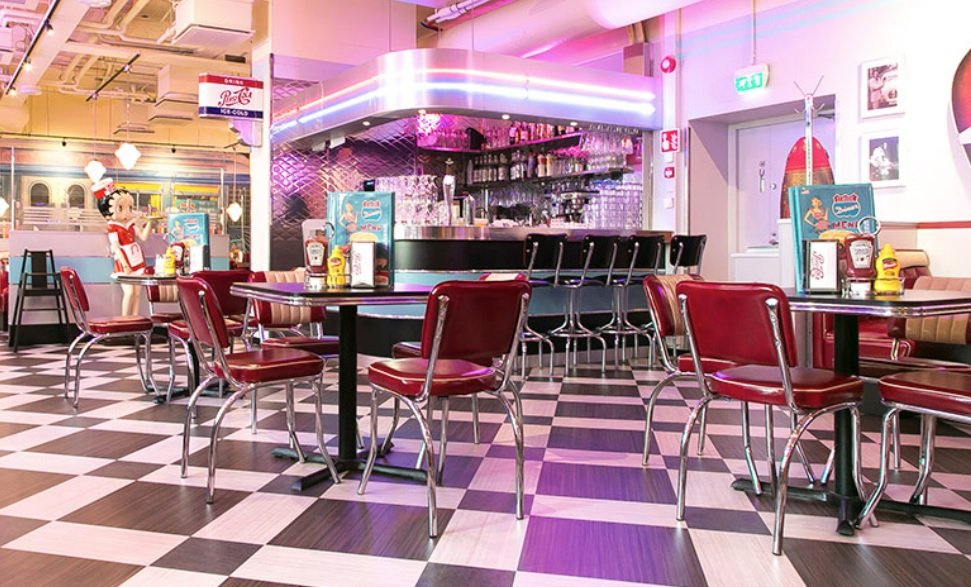The photograph showcases a vibrant, retro-style diner reminiscent of the popular 50s and 60s era, complete with a black and white checkered floor. Prominently displayed on the left-hand side is a large plastic caricature of Betty Boop in a red dress, holding a tray. The diner is populated with numerous tables, each with a black top and a single stem base, surrounded by chrome-legged red leather chairs. Every table is neatly set with a blue menu, featuring a road sign design in the top corner, along with condiments such as ketchup and mustard, and napkins. In the background, there is a bar area with metallic-based black stools, and neon lighting illuminating the space above it. The ceiling adds an industrial flair with exposed piping. Additionally, a Pepsi-Cola sign is hanging to the left, contributing to the nostalgic decor.